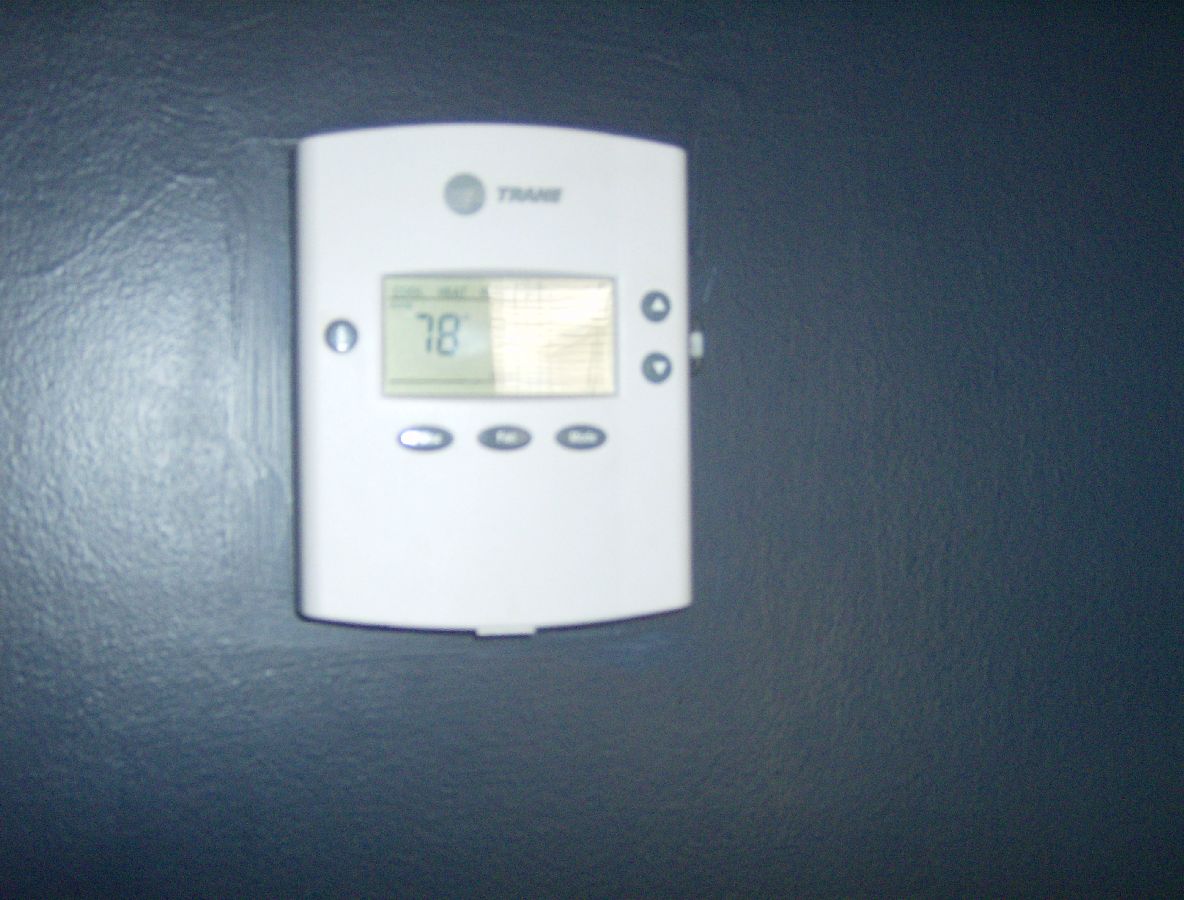A blurry and low-quality photograph appears to have been taken with a flash, as evidenced by the light reflecting off the navy-colored painted wall behind the subject. The image focuses on a white thermostat that stands out prominently against the dark backdrop. Despite the blurred focus, the thermostat displays a clear temperature reading of 78 degrees. The brand logo on the device seems to vaguely spell out "T-R-A-S" or possibly "T-R-A-E." Encircling the temperature display are several dark gray buttons. To the right of the display, there are up and down arrow buttons, and at the bottom, there are three indistinct buttons whose functions are not readable. On the left side, there's a single circular button. The thermostat itself is rectangular with rounded top and bottom edges, adding a slight touch of design to its functional appearance. The temperature display area is a pale green color, providing a subtle contrast to the overall white and gray color scheme.